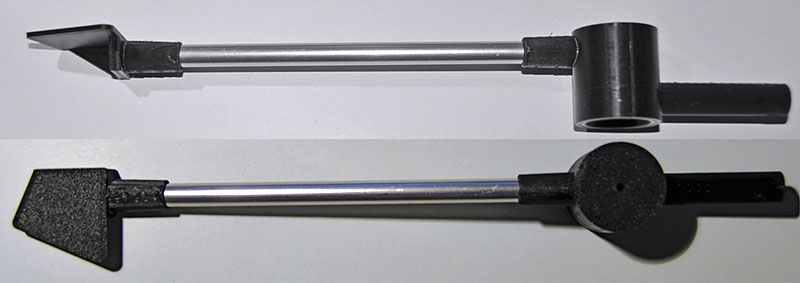This detailed caption combines the information from all three descriptions:

The image is divided into two sections, each depicting a black and white photograph of a long, thin tool, each picture oriented differently. The top photograph shows the tool from a side view, while the bottom photograph presents an overhead view. The tool itself features a long metal rod attached to a tubular hollow tube, extending horizontally from left to right.

On the left end, there is a black plastic piece, angular and flat on top. This resembles a sprayer tip with a smaller plastic cover. The middle section is a silver bar, and the right side of the tool has a black handle-like shape with three plastic cylinders, presumably for gripping. The tool’s design indicates it may be a sprayer, with attachments and a nipple to connect additional hoses. The background of both photographs is light blue, and the overall layout of the photographs is much wider than it is tall.